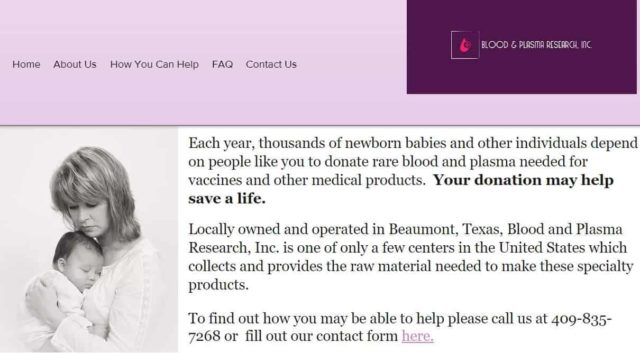The image is a screenshot of a women's healthcare website. At the top left of the page, there are navigation links for 'Home,' 'About Us,' 'How You Can Help,' 'FAQ,' and 'Contact Us.' On the right side of the screen, the website is branded with the name "Blood and Plasma Research Inc." 

The main text centered on the page reads: "Each year, thousands of newborn babies and other individuals depend on people like you to donate rare blood and plasma needed for vaccines and other medical products. Your donation may help save a life. Locally owned and operated in Beaumont, Texas, Blood and Plasma Research Inc. is one of only a few centers in the United States that collects and provides the raw materials needed to make these specialty products. To find out how you may be able to help, please call us at 409-835-7268 or fill out our contact form here." The word 'here' is highlighted in lavender for emphasis.